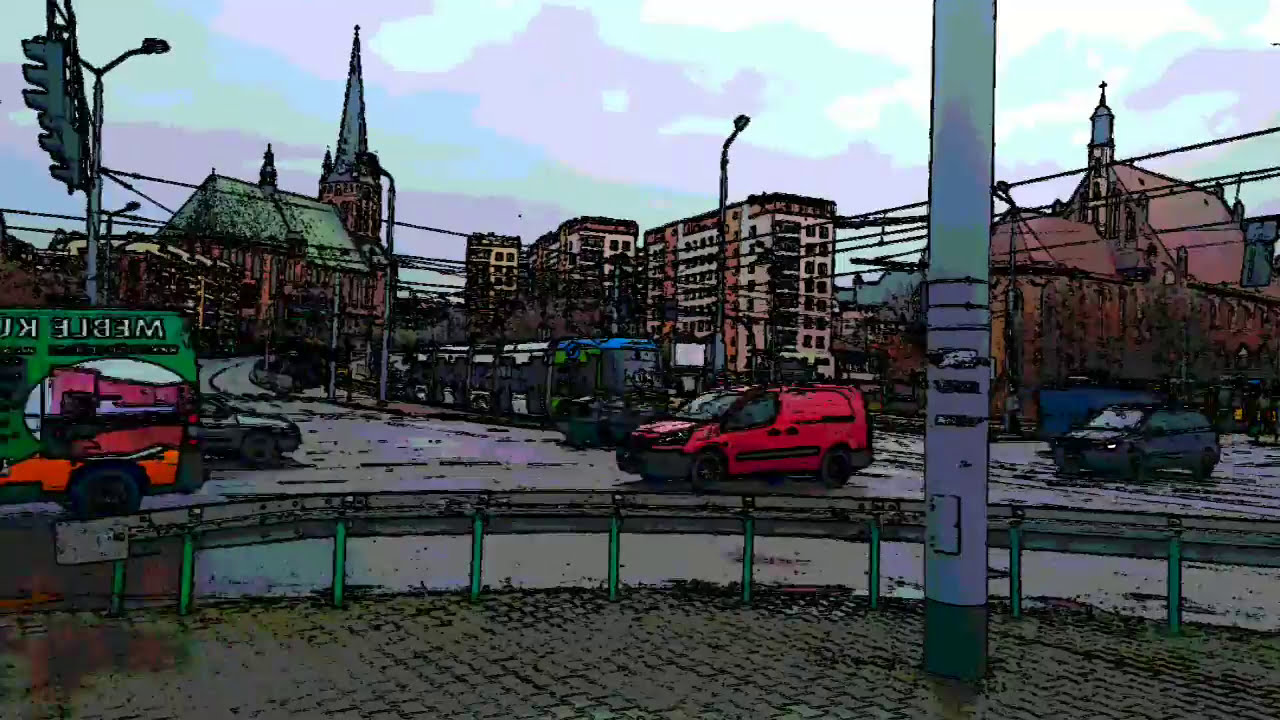This detailed, richly colored image depicts a city street, rendered in a cartoon-like, watercolor style, possibly enhanced with a Photoshop filter to achieve its distinctive look. In the foreground, a pole and a fence border a road lined with several parked vehicles, including a red car, a red van, and a black minivan. A street lantern and traffic lights add to the urban scene. To the left side, a red traffic light hangs above a structure with an illegible inscription, potentially reading "M-E-B I-L." Several buses are parked in the mid-ground, with a prominent brown church, featuring greenish steeples, standing just behind them. To the right of the church, three high-rise buildings with numerous windows form a rectangular, gray or white backdrop. Further to the right stands another church with a smaller steeple and a gabled roof adorned with a cross. In the far background, the sky displays a dynamic mix of purple, blue, and greenish hues, reinforcing the overall lively yet gritty atmosphere of the city. Although devoid of people, the scene conveys a sense of urban motion and life, with a mixture of transportation modes including a streetcar or tram, enhancing the European city ambiance.